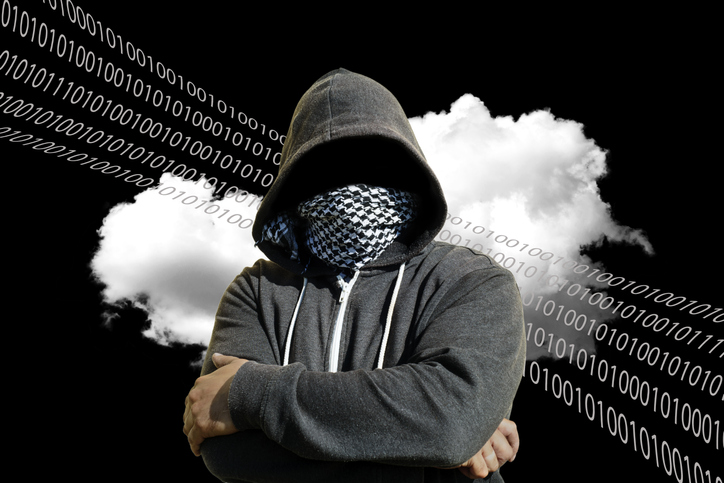This photograph is a heavily stylized and edited image predominantly in shades of gray, black, and white. Central to the image is a man standing with his arms crossed over his chest. He is wearing a gray zip-up hoodie with a white zipper and drawstrings, with the hood pulled up, casting a shadow over his face. His face is entirely obscured; the top half hidden in shadow and the lower half covered by a black and white checkered bandana. His light-colored hands, which appear to be Caucasian, hold his arms. The background is black, featuring a dense, white cloud-like plume centrally placed, resembling an edited explosion. Overlaying this background are five descending rows of binary code, "10101010," stretching diagonally from the upper left to the lower right corner. The interplay of elements and the concealed identity of the individual suggest an image of a hacker or someone associated with the dark web.